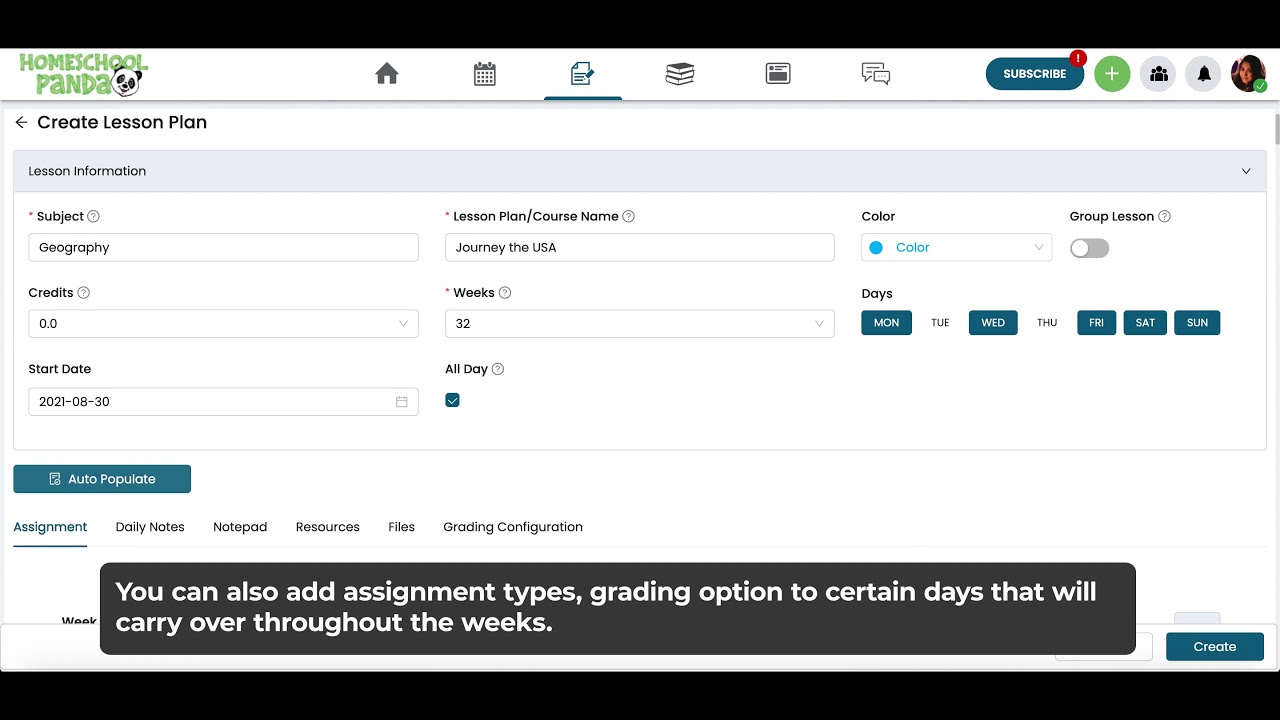This is a detailed screenshot of the "Homeschool Panda" website. The interface displays several navigational tabs, each represented by distinct icons: a home tab, a calendar tab, a document tab, a tab resembling a book, another tab with a card-like icon, and a chat tab. 

At the top of the page, there are several buttons including one for subscribing, another one labeled 'Press', an icon button, a bell icon, and a circular profile picture of a girl, which likely represents the user. 

The main section of the screenshot features a section for creating a lesson plan with detailed fields and inputs. The lesson information includes:
 
- **Subject**: Geography
- **Lesson Plan/Course Name**: Journey v. USA
- **Credits**: To be possibly input or adjusted
- **Weeks**: 32 weeks
- **Start Date**: 2021-08-30
- **All Day**: This option appears to be selected

Additionally, there is functionality for auto-populating certain data and fields to add assignment types, grading options, and specific days that will be carried over throughout the weeks.